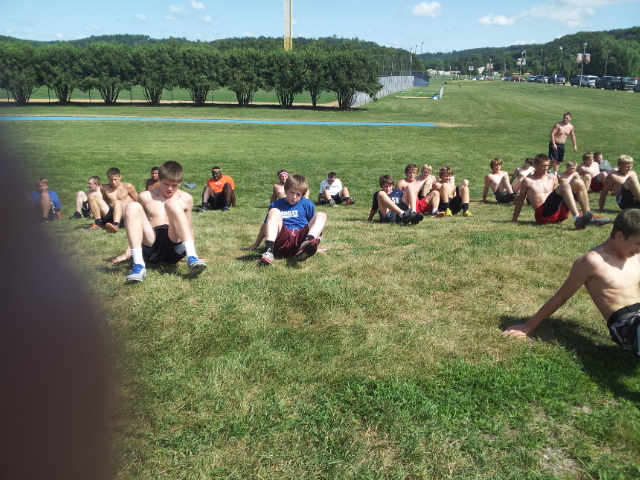In this vividly captured photograph, approximately 20 young boys, varying in age from early to late teens, are gathered on a grassy field. Most of them are sitting on the ground, propping themselves up with their hands behind them, and bending their knees as if in a crab-walking position. They are dressed in athletic attire, primarily gym shorts and a mix of T-shirts and bare torsos. The boys are directed towards the camera, with one standing among them.

The scene is set against a backdrop of a light blue sky adorned with low-hanging clouds. A row of trees lines the distance, contributing to the scenic, park-like ambiance. To the right, a series of streetlights and a collection of parked cars are visible, alongside a chain-link fence that suggests the proximity of a recreational area, potentially a soccer or baseball field. Additionally, two African-American men are positioned at the back, overseeing the group, adding a sense of supervision or coaching to the moment captured.